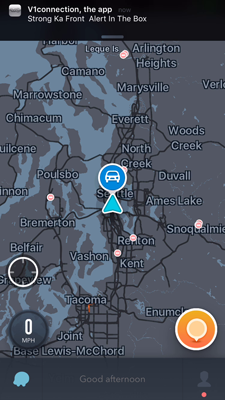This is a detailed description for the caption provided for the screenshot:

---

**Map Screenshot from a Mobile Application**

This screenshot from a phone displays a map interface with a variety of elements and notifications. 

- **Top Section:** The top inch and a half of the image features a black border. In the left corner of this border, there's a silver square. To its right, in silver text, it reads "V1 Connection, the app". Just barely visible in faded silver text, it says "Now". Below that, it reads "Strong Ka Front Alert" within a highlighted box.

- **Map Area:** The main portion of the screenshot is a map. The left edge of the map displays a small water body shaded in light blue, which extends midway down and continues off the left side about two inches from the bottom. The land mass is rendered in dark gray. At the center of the map, there's a blue circle with a white border containing a white car icon. Below this car icon is a light blue triangle with a white border.

- **Roads and Labels:** The roads are delineated with black lines, while their names are labeled in white text throughout the map.

- **Bottom Right Corner:** In the bottom right corner of the map, there's an orange circle with a white border, containing a smaller white circle inside it. Adjacent to this on the left is a black circle with white text reading "0 MPH."

- **Scope-like Icon:** Above the orange circle, there's a scope-like icon in white with a black border, giving the appearance of a crosshair.

- **Bottom Section:** The last inch of the screenshot features a dark gray border. In the center of this border, in light gray text, it says "Good afternoon." On the left side, there is a blue emblem resembling a pea (suggesting a bank emblem). On the right side, there is a human head icon with a red dot underneath it.

This descriptive caption captures the various components and visual layout of the map screenshot, providing a clear and detailed understanding of the image.